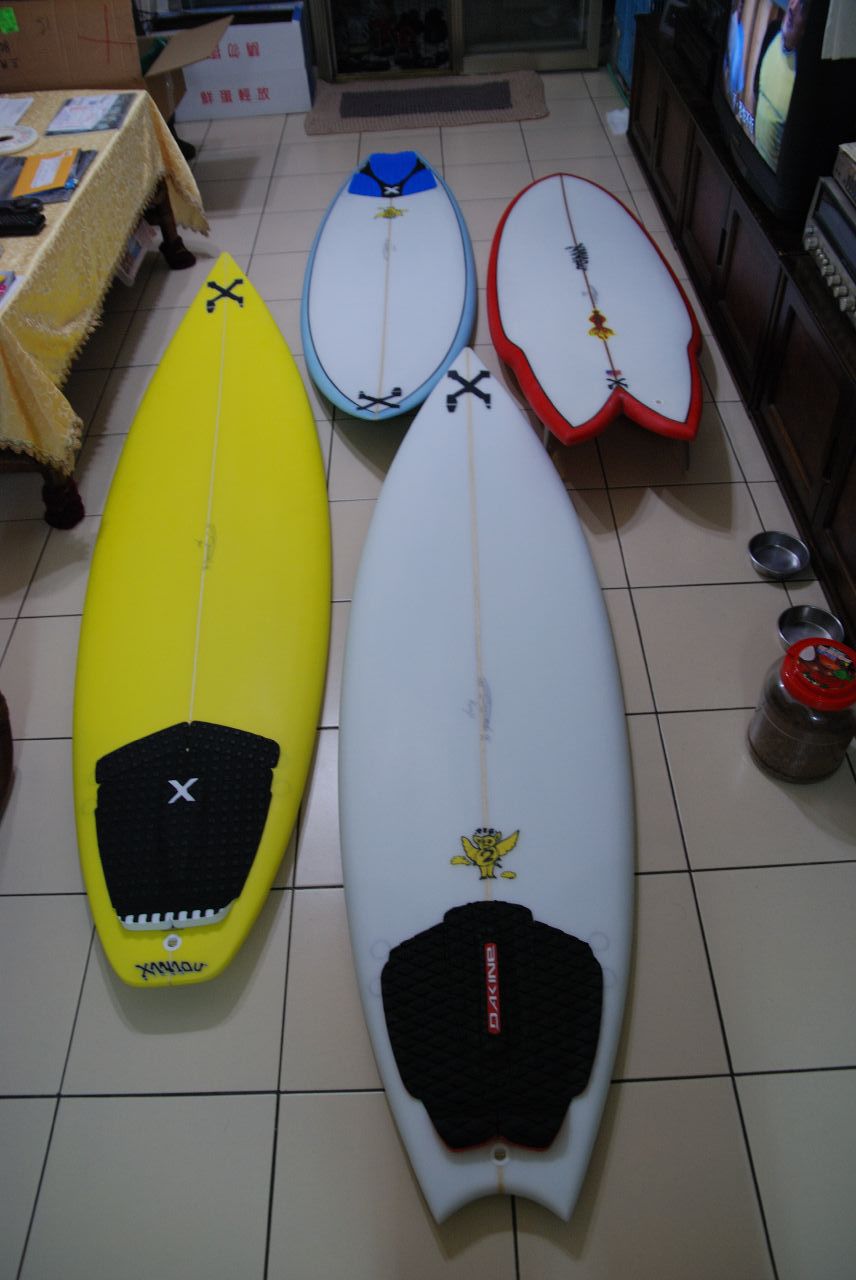In this color photograph shot in portrait mode, we see a domestic living area with tan-colored tile flooring and black grout. At the center of the image are four boogie boards laid out on the floor. The boards include a long yellow one with black accents, a long white one with a yellow icon featuring a winged character, a shorter white board with a blue border and "X" icon, and another shorter white board with a red border.

On the right side of the floor, two metal pet food dishes are positioned next to a glass jar with a red lid, presumably holding pet food. Adjacent to this setup, a dark wooden cabinet supports an active television set. At the image's left, there is a brown wooden table dressed with a yellow tablecloth that has a fringed edge, cluttered with various items including some mail. A door is visible in the top center of the image, complete with a doormat in front of it. The overall scene captures a casual and functional living space with an eclectic mix of items and color.